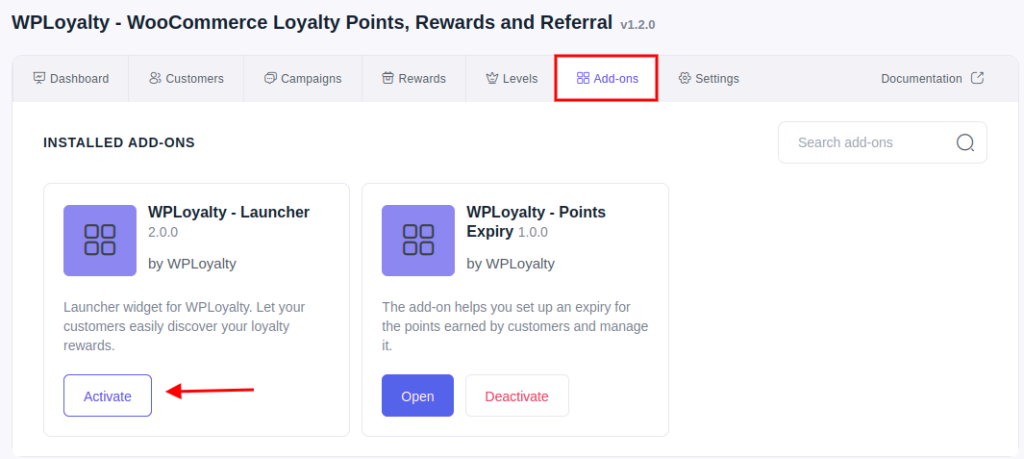This screenshot showcases the interface of the WPLoyalty plugin within WooCommerce, specifically highlighting the "Loyalty Points, Rewards, and Referral" section. The interface is enclosed in a gray box and features tabs labeled Dashboard, Customers, Campaigns, Rewards, Levels, Add-ons, Settings, and Documentation.

The Add-ons tab is selected and highlighted in red, indicating it is the active section. Within this tab, there is a subsection titled "Installed Add-ons" that lists the currently installed features:

1. **WPLoyalty Launcher 2.0 by WPLoyalty**: This add-on includes a launcher widget designed to help customers easily discover their loyalty rewards. A red arrow points to the "Activate" button, signifying that this add-on can be activated.

2. **WPLoyalty Points Expiry by WPLoyalty**: This add-on assists in setting up an expiry date for the loyalty points earned by customers, allowing for efficient management of these points. The options for this add-on include a blue "Open" button for configuring the settings and a white "Deactivate" button highlighted in red for disabling the feature.

Overall, this screenshot effectively illustrates the add-ons available within the WPLoyalty plugin, along with their respective activation and management options.